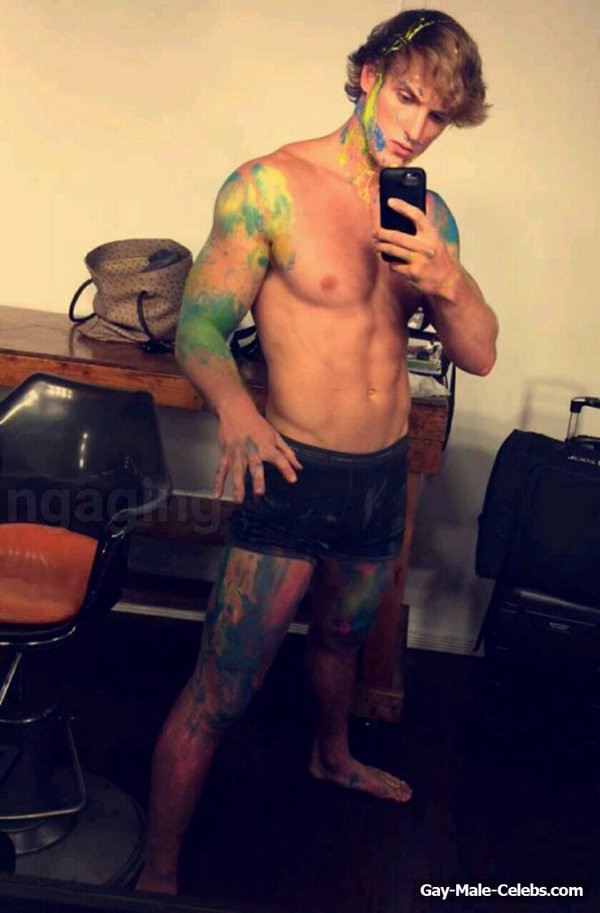In this detailed photographic image taken indoors, a young, muscular white man with shaggy, medium-length blonde hair, reminiscent of an old-style Justin Bieber haircut, stands barefoot. He is shirtless and clad only in black swim trunks or boxer briefs. His arms, shoulders, and legs are adorned with intricate yellow and green markings that could be mistaken for tattoos but appear to be paint. Some blue and additional green paint is splattered across his elbows, knees, face, and even a bit in his hair. The young man, possibly one of the Paul brothers (Jake or Logan), is engrossed in his smartphone, capturing a selfie with a black phone, his face focused in concentration. To his right is a piece of luggage with a handle standing in as a makeshift chair, and to his left is a desk holding a brown purse, alongside an orange-upholstered office chair. The wall behind him is an off-white or beige, creating a neutral backdrop. A noticeable watermark at the bottom right corner of the image reads "gay-male-celebs.com."